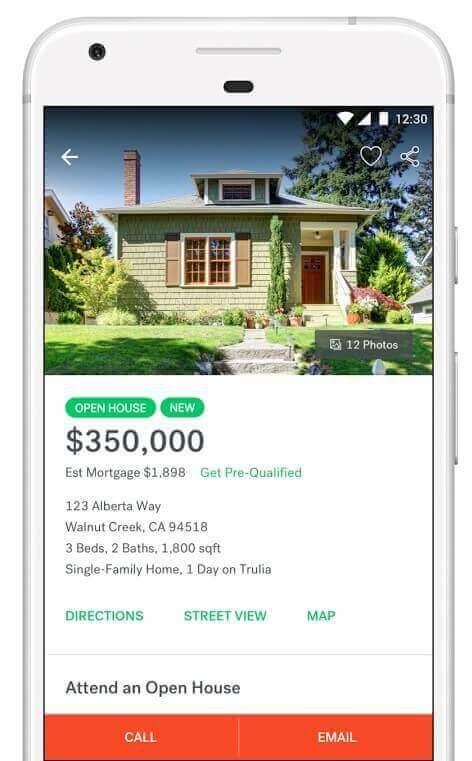A vertical rectangular image of a white cell phone captures the top two-thirds of the device. The cell phone's screen displays a real estate listing. In the top portion of the screen, there's an image of a small house set against a gradient blue sky that darkens towards the top and lightens towards the bottom, where fluffy white clouds are visible. The house has a dark front door, a green lawn, and two concrete steps leading up towards the center, followed by additional steps leading up to the door. Trees are planted along the front of the house.

In the upper right-hand corner of the screen, there is an outlined heart that isn't filled in yet. In the upper left corner, there is a left-pointing arrow. Below the house image, two horizontal green ovals with white capital letters are displayed. The larger oval on the left reads "OPEN HOUSE," while the smaller oval to the right reads "NEW."

Further down, bold black font shows the price "$350,000." Below this, in regular black font, it states "EST mortgage $1,898" and then in green "Get pre-qualified." Continuing in black regular font, the address is listed as "123 Alberta Way, Walnut Creek, CA 94518." Additional details include: "3 beds, 2 baths, 1,800 SQFT," followed by "Single-family home, 1 day on Trulia."

Towards the bottom, green uppercase letters state "DIRECTIONS," with adjacent options "Street View" and "Map" to the right. Below this, black bolded font reads "Attend an open house."

At the very bottom of the screen, an orange horizontal rectangular area is divided lightly by a white line. The left side of this area has white uppercase font that says "CALL," and the right side says "EMAIL."